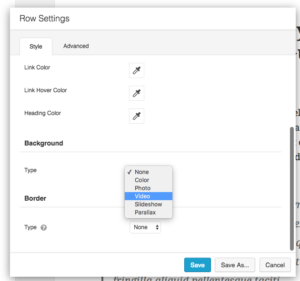In this image, we observe a compact settings menu that appears to belong to a mobile device, likely a phone or tablet, though it could potentially be a desktop interface. The menu is displayed against a white background. At the top, the heading reads "Row Settings." Directly beneath that, there are two tabs labeled "Style" and "Advanced," with the "Style" tab currently active.

Within the "Style" tab, several customization options are listed. The first option is "Link Color," followed by "Link Hover Color," and then "Heading Color." Next, there is an option for "Background," which is succeeded by "Type," "Border," and another "Type" with a question mark beside it for further details.

Below these options, there is an open dropdown box, which seems to be scrollable, most likely for selecting the "Border Color" as the "Border" option is highlighted. Choices within this dropdown include "None," "Video," "Slideshow," "Parallax," and "Photo."

At the bottom of the menu, three buttons are visible: "Save," "Save As," and "Cancel," allowing the user to save their settings, save them under a new name, or cancel their changes, respectively.